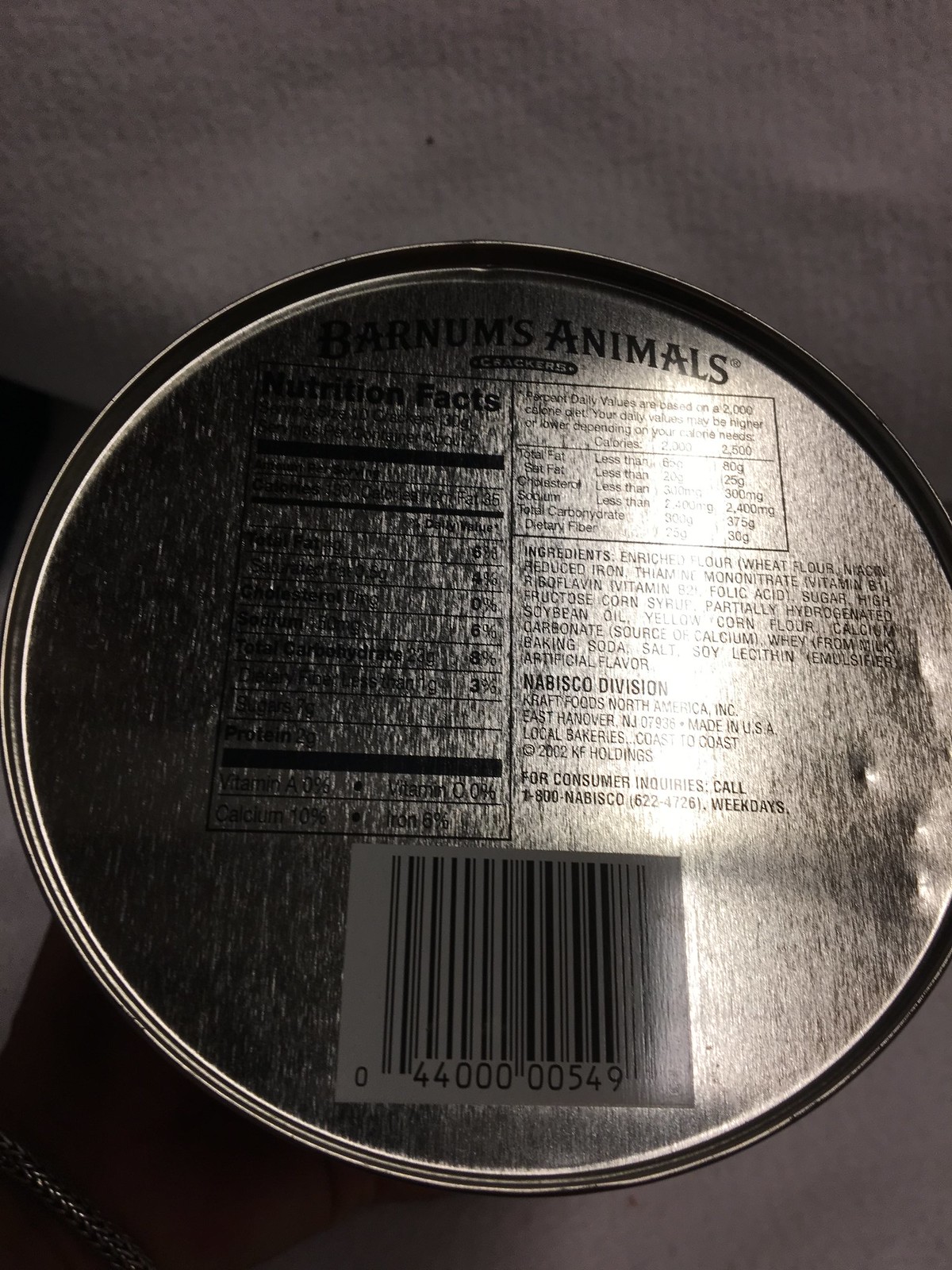The photograph captures the back of a shiny, circular aluminum tin prominently displaying the brand name "Barnum's Animals" at the top. The reflective surface makes details challenging to discern, particularly on the right side where sunlight causes a noticeable glare. Visible on the tin are sections labeled "Nutrition Facts" and "Ingredients," though the details are hazy due to the brightness. Some of the legible ingredients include wheat flour, corn syrup, and enriched flour, framed within a white square containing small black lines. The background consists of a bumpy white cloth, and at the bottom left, a hand adorned with a silver bracelet holds the tin. The bottom of the tin, with indentations and a barcode, further suggests it could be the lid of an animal cracker container, indicated by partial wording and context clues.